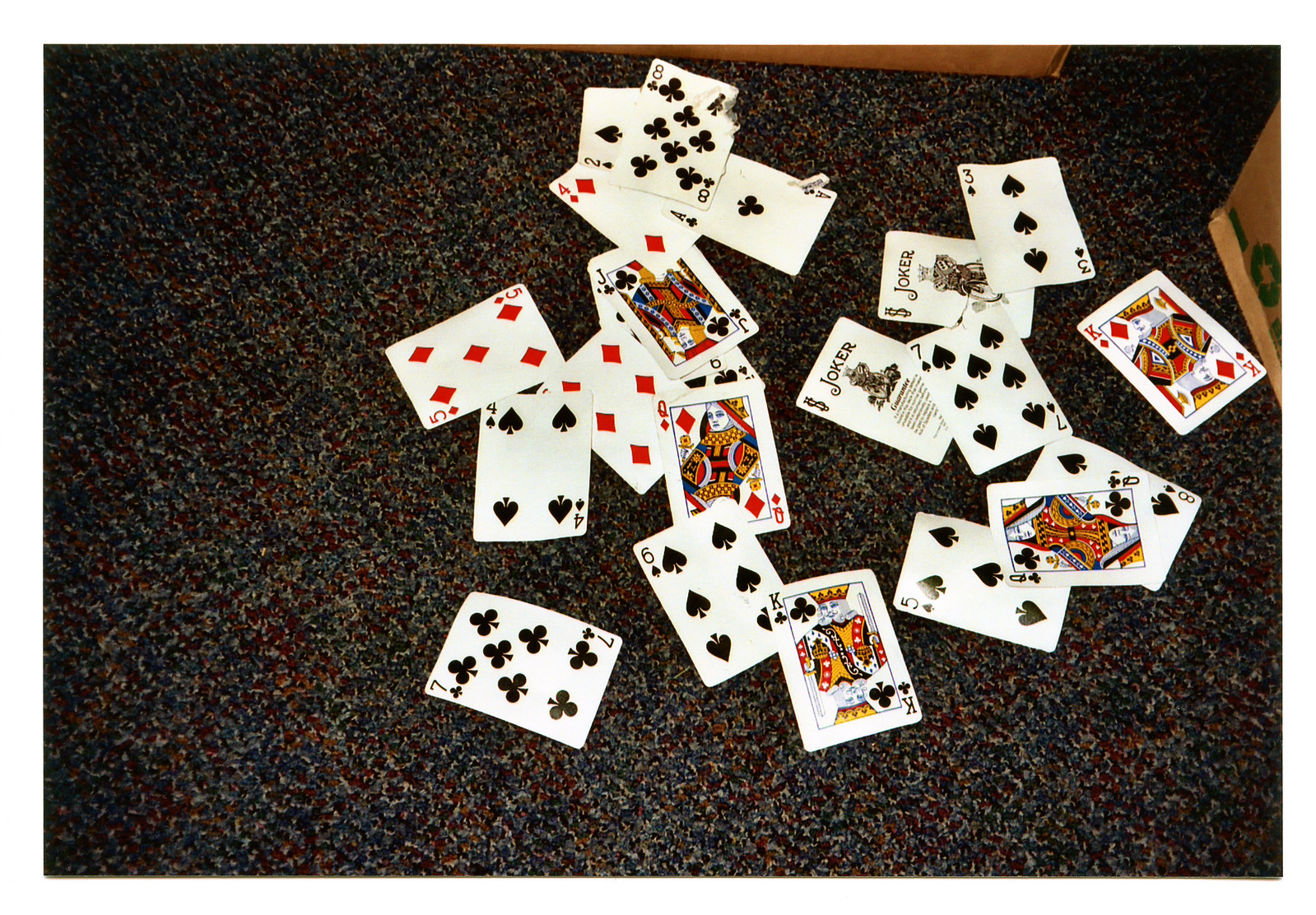In the image, a scattered assortment of playing cards lies on a red and white industrial carpet, the type commonly found in hotel rooms. The carpet, featuring red, blue, and white hues, is low-pile and durable. Among the cards, which form a partial deck, both jokers are visible. The cards appear haphazardly thrown across the floor, and many show signs of wear, with some bent and others having water damage. Notably, the eight of clubs card appears to be either burnt or torn. To the right of the cards, a small, upside-down cardboard box can be seen, measuring approximately four inches horizontally and three inches vertically. The box features a visible green recycling symbol with arrows. The focus of the image is primarily on the discarded cards against the backdrop of the distinctive carpeting.